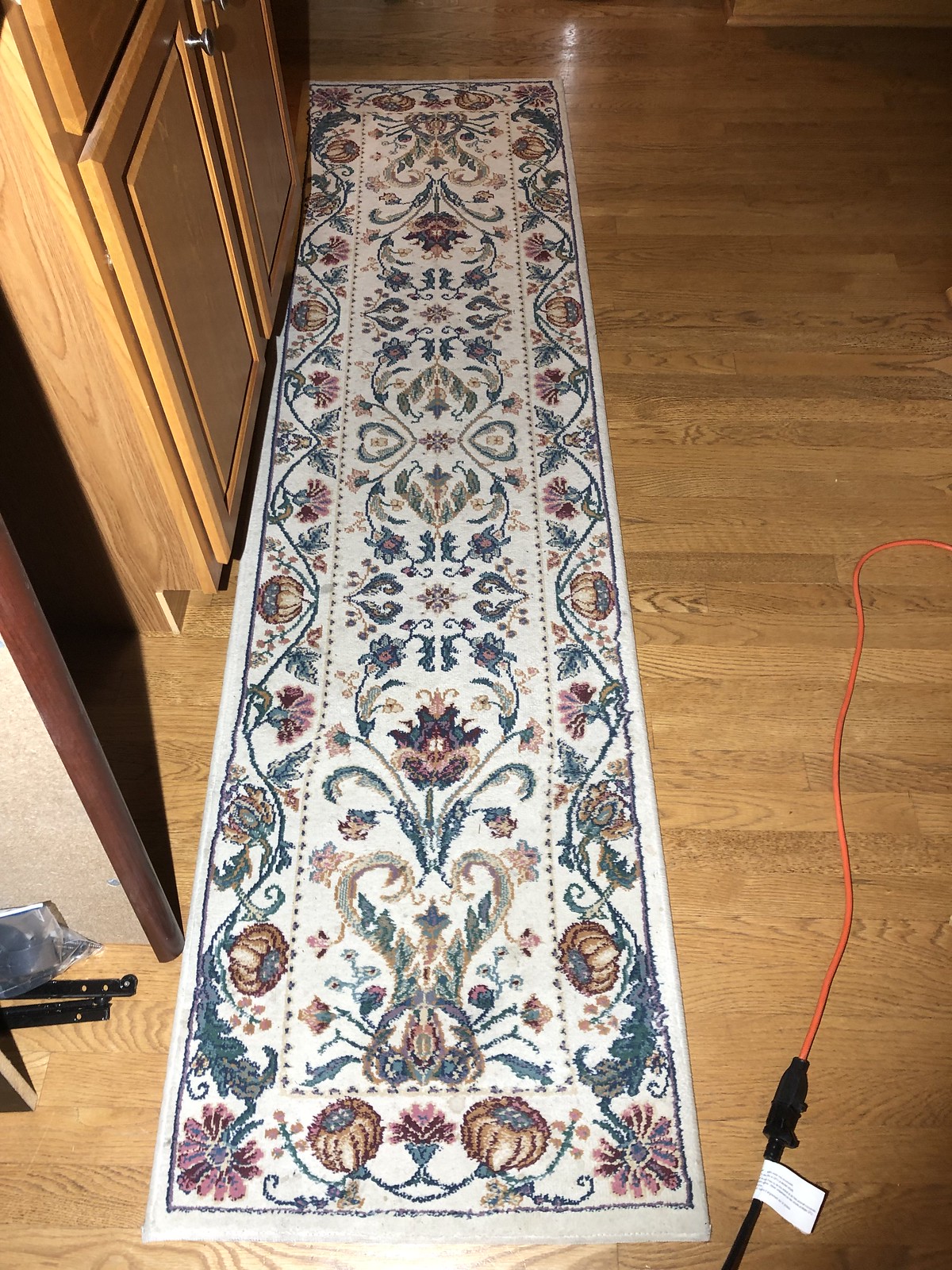In this detailed photograph of a room, we see an interior space with a natural wood floor. On the left side of the image, there is a wooden cabinet, matching the floor’s brown hue, featuring two doors with silver knobs, and a drawer or additional cabinet space above. The focal point of the image is a long, narrow area rug, measuring approximately 6 to 8 feet in length and 15 to 18 inches in width, adorned with a traditional floral pattern on a beige background with accents of green, turquoise, pink, and burgundy. To the right of the rug, an orange extension cord is connected to a black extension cord with a white label and a black switch. In the upper left corner, there appears to be a small opening that could be part of a closet, containing black racks and a plastic bag filled with nuts, bolts, and shelf components. The overall setting gives a warm, rustic feel to the room.